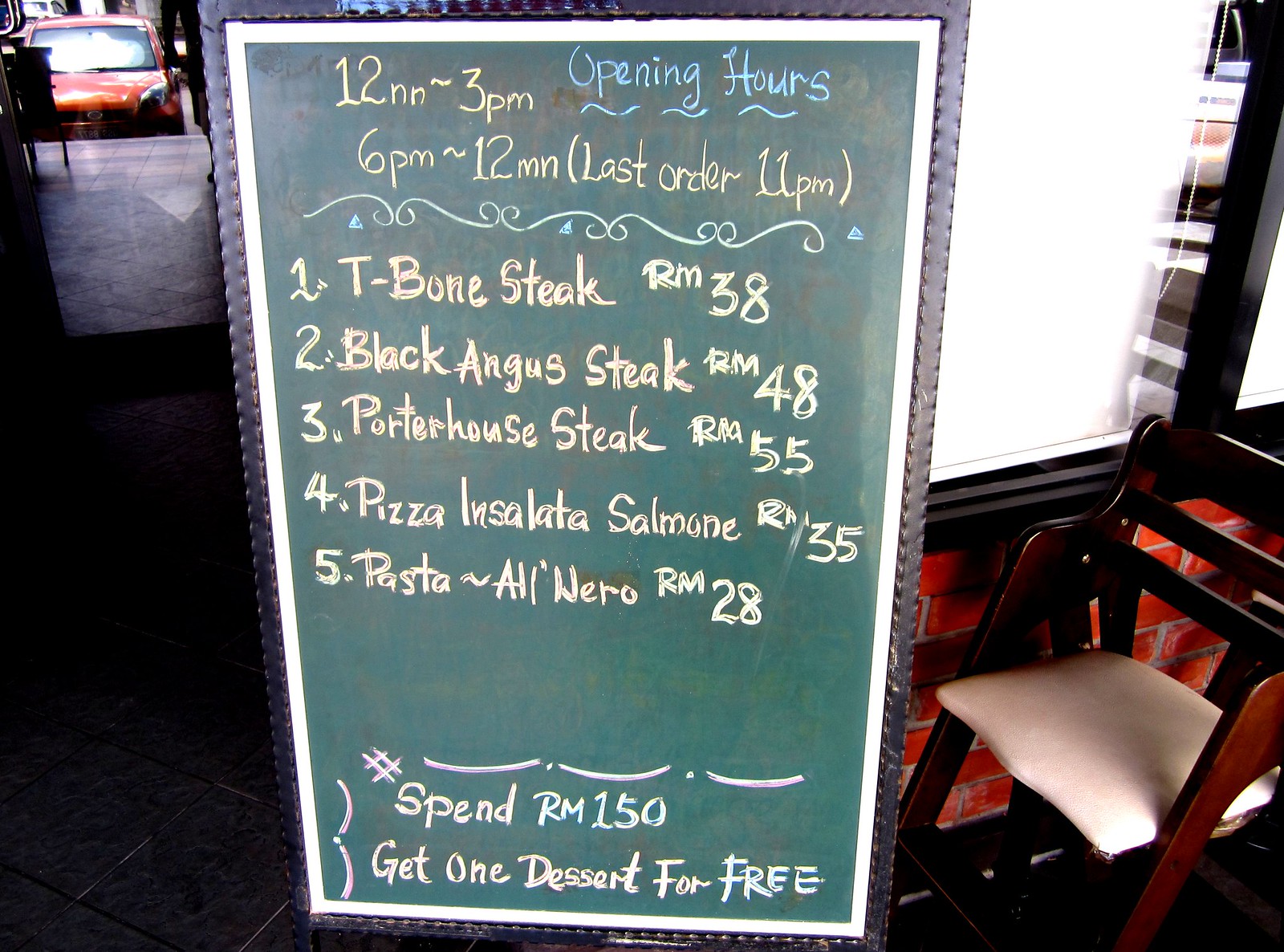The image displays a large rectangular chalkboard sign outside a restaurant. The chalkboard, framed by a rustic purple twisty frame, has a turquoise background. Written in light blue chalk at the top are the opening hours: "12 p.m. - 3 p.m." and "6 p.m. - 12 a.m. (last order at 11 p.m.)." The menu lists five items: "1. T-bone steak - RM38, 2. Black Angus steak - RM48, 3. Porterhouse steak - RM55, 4. Pizza and Salata Salmon - RM35, 5. Pasta a la Nero - RM28." At the bottom, there's an offer that reads "Spend RM150, get one dessert free," indicated by a hashtag/pound symbol. To the right of the chalkboard, a small wooden chair with a white cushion is placed next to a brick wall. On the left, you can glimpse a doorway or window opening up to a parking lot.